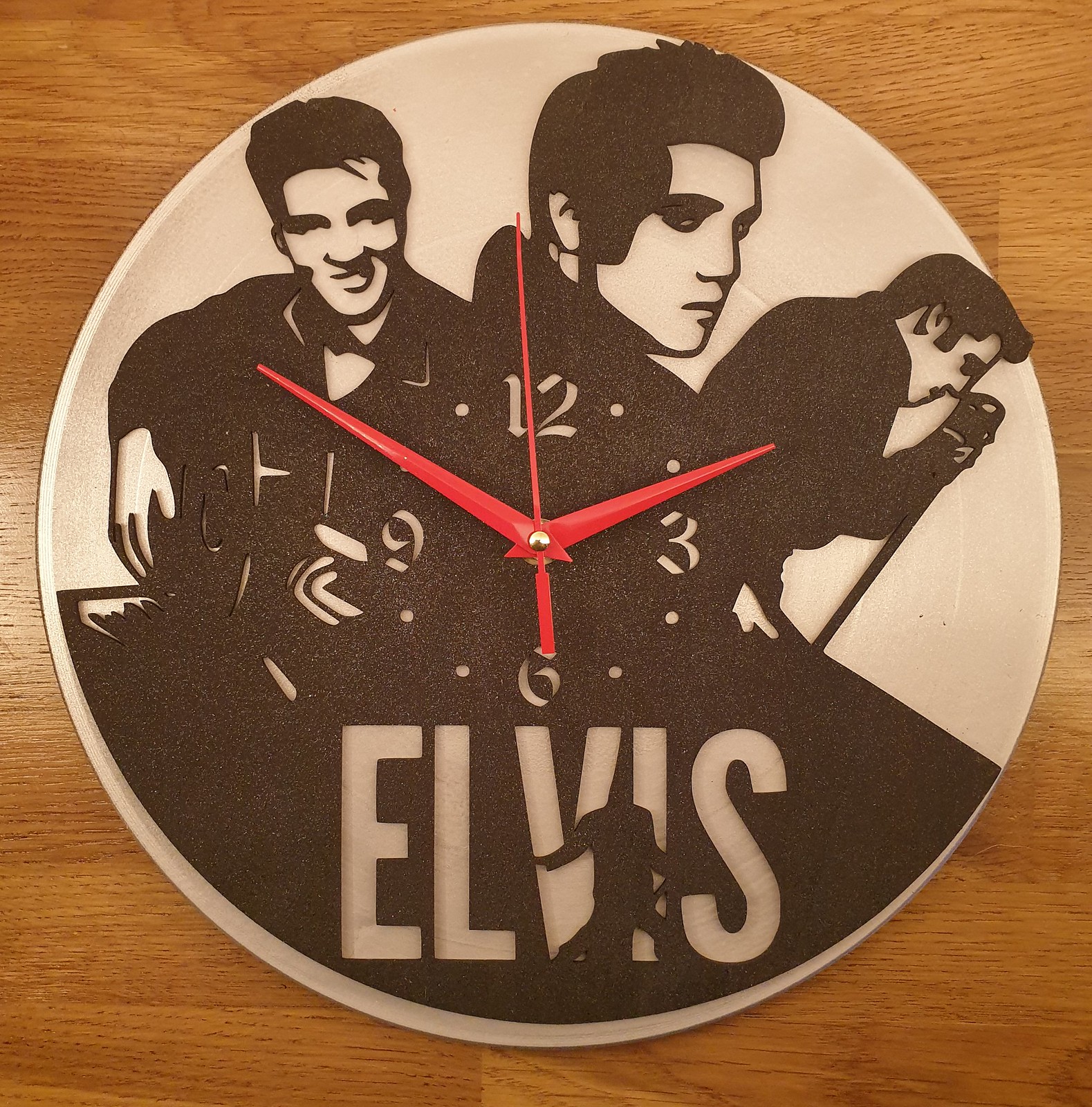The image features a striking 3D printed clock set on a basic brown wooden surface, resembling an oak floor or table. The clock's design mimics a vintage record and showcases three black and white depictions of Elvis Presley. To the left, Elvis is strumming a guitar and smiling; in the middle, he strikes a somber pose with his collar turned up; and on the right, he is passionately singing into a microphone. The clock's face is light tan with dark brown cutouts and includes the numbers 12, 3, 6, and 9 in a small central circle, with dots marking the remaining hours. Red, modern-looking hour, minute, and second hands add a vibrant touch. At the bottom of the clock, the word "Elvis" is displayed in light beige letters, featuring a subtle black silhouette of Elvis within it, making it a unique tribute to the legendary musician.